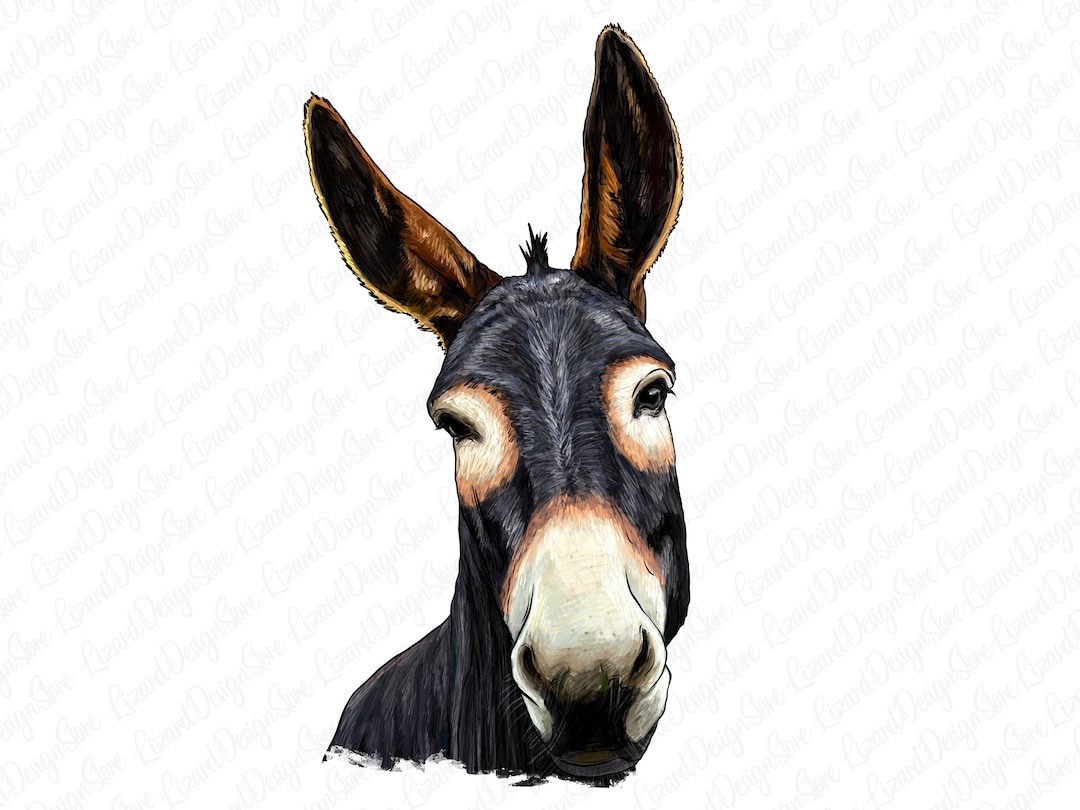The image is a square, multi-colored artistic piece of a realistic looking black donkey, or possibly a mule, depicted in either a painting or colored pencil artwork. The donkey is facing directly at the viewer, capturing attention with its expressive gaze. Its ears, which are long, brown, and fuzzy, stand upright atop its head. A distinctive tuft of black hair reminiscent of an alfalfa sprout protrudes from the middle of its head. The donkey’s black body contrasts with its white snout and the white patches around its black eyes, which are accentuated with a red ring around the white portions. The background of the image is the white of a computer screen, prominently featuring a repeated diagonal watermark that reads "Lizard Design Store."